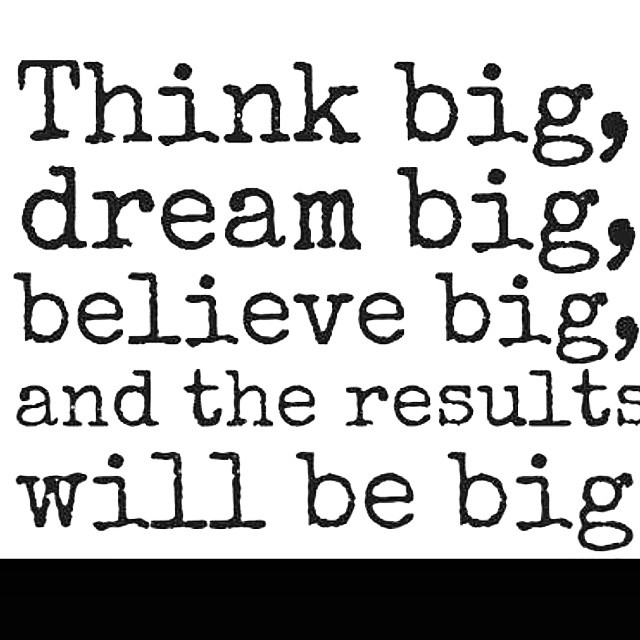The image features a bold statement in large black text against a stark white background, utilizing a typewriter-style font. The text reads, "Think big, dream big, believe big, and the results will be big." This message, presented in five lines, dominates approximately 95% of the image. Below the motivational quote, there is a solid black rectangular border, which serves to underscore the statement. The overall composition resembles a screenshot or a meme, with the distinct impression of handwritten or typewritten text, though clearly formatted in a digital typewriter font. The simplicity of the design, with its black and white contrast, emphasizes the powerful and inspirational message.